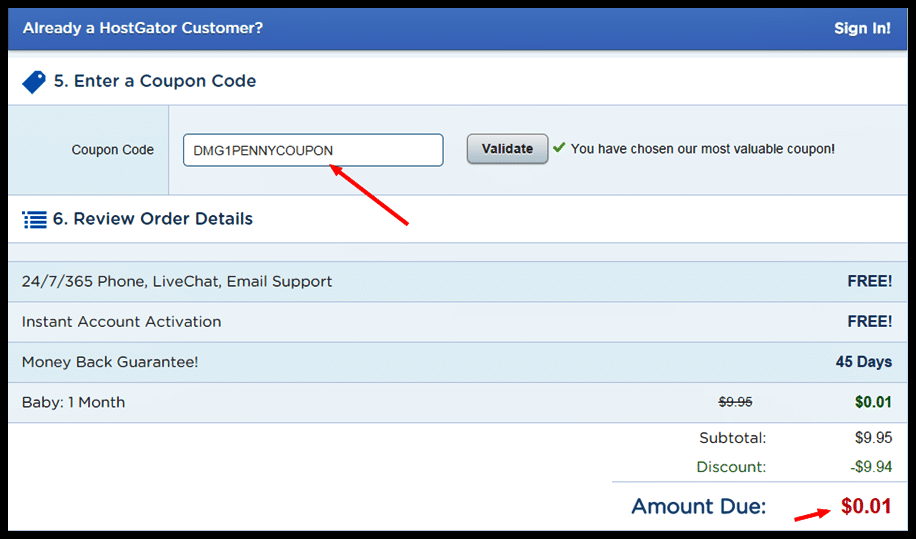The image is a screenshot from a webpage displaying a HostGator promotion. At the top of the page, a blue bar reads "Already a HostGator customer? Sign in." The word "HostGator" is clearly spelled out as H-O-S-T-G-A-T-O-R. Below this bar, there is a blue icon resembling a coupon with the number five next to it. The text next to the icon instructs users to "Enter a coupon code," followed by a field labeled "Coupon Code." The specific coupon code shown is "DMG1PENNYCOUPON," which is highlighted with a red arrow pointing towards it for emphasis.

At the bottom of the screenshot, the pricing details are displayed. The total amount due is prominently shown as $0.01, with a red arrow emphasizing this price. The breakdown reveals an initial subtotal of $9.95, which is located in the bottom right-hand corner. A discount of $9.94 is applied, resulting in the final amount due of $0.01. The image also includes miscellaneous sections of the webpage in the background, providing additional context.